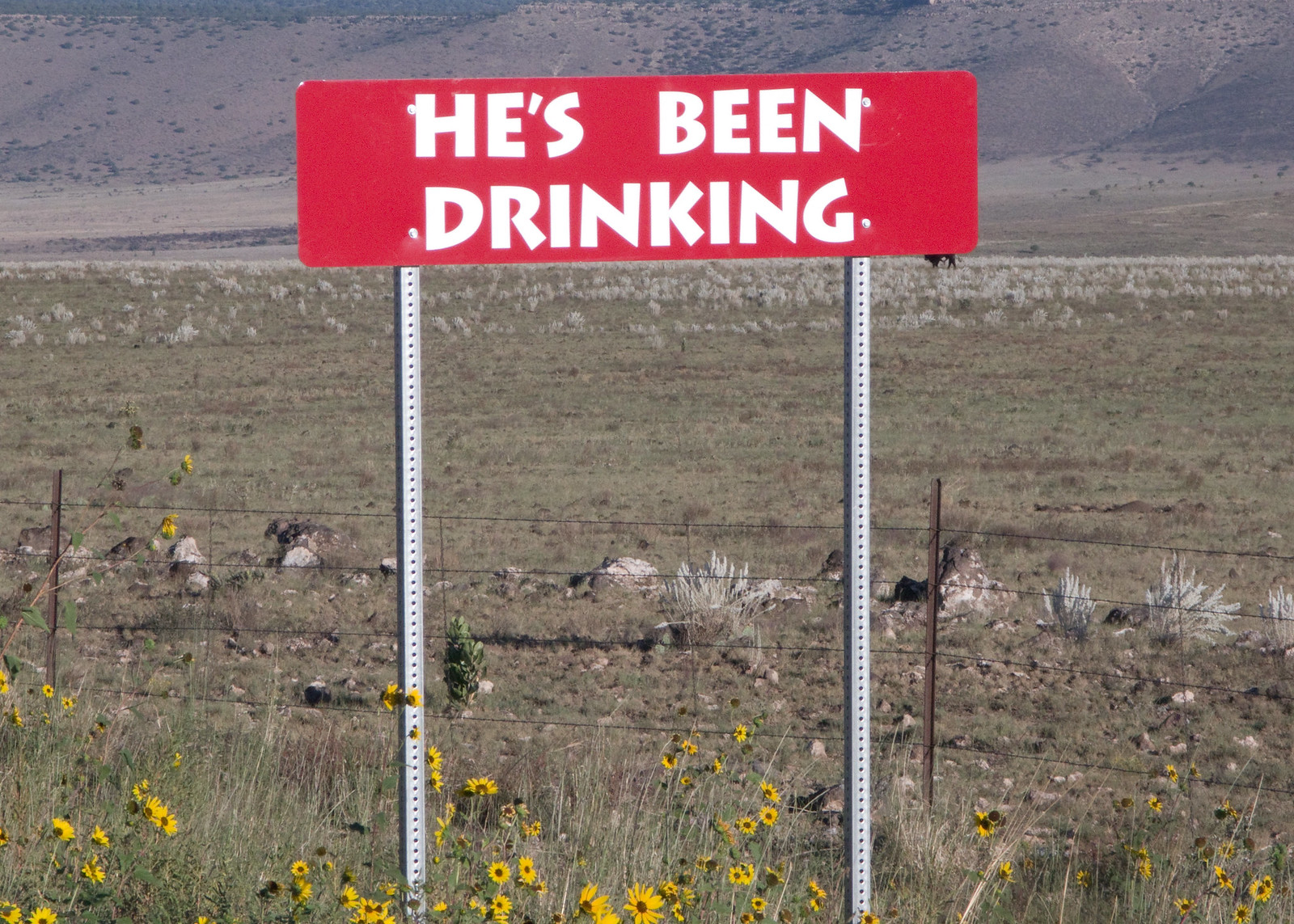This vibrant color photograph captures a rectangular red sign held aloft by two tall metal poles on either side. The sign features white text that reads, "Ead's been drinking." The setting appears to be outdoors amidst a natural landscape.

Beneath the sign, there's a patch of green grass adorned with yellow flowers, some boasting a black center. Directly behind the sign, a fence made of thin black poles and wiring adds a rustic element to the scene. 

The middle ground transitions to a more beige and faded expanse of grass, interspersed with clusters of beige or white-leaved plants. In the distance, a breathtaking mountain range, composed of varying shades of grey, serves as the photograph's backdrop. 

The whitish plants increase in density as they approach the mountains, enhancing the composition's depth. Notably, two small clumps of yellow flowers peek out from behind the fence on the left side, while the majority of these flowers are situated directly below the sign, adding a pop of color to the serene landscape.